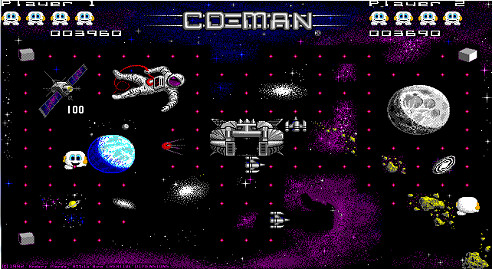The image is a vibrant screenshot from a retro-style video game set in outer space. The background is predominantly black, speckled with patterns of multicolored dots — pink, purple, and blue — replicating the look of distant stars. A distinctive line of purple stars is grouped prominently in the scene.

On the left side of the image, an astronaut figure drifts towards the center, navigating through an environment populated with various celestial objects like planets and asteroids. Among these, there is a peculiar smiling face with blue eyes and a yellow outline.

At the top of the screen, the game's HUD (Heads Up Display) indicates game information. "Player One" is represented by small white icons with blue eyes, symbolizing their remaining lives. Similarly, "Player Two" is marked by identical icons. Both players' scores are displayed beneath their lives count. The title of the game, "CDEMAN," is visibly inscribed at the top, adding a nostalgic touch to the overall aesthetic of the game.